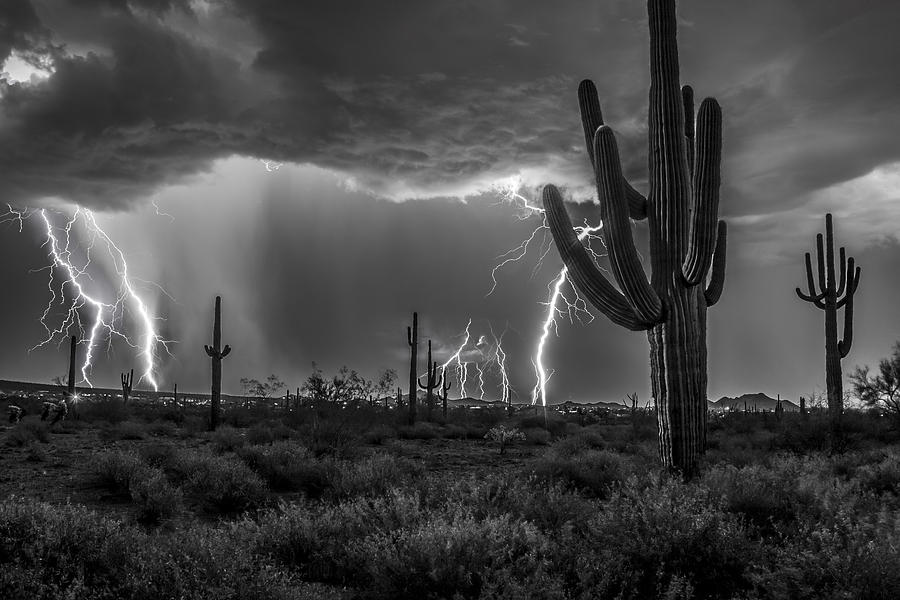This black and white photograph captures a dramatic desert scene in the midst of a lightning storm, likely taken at night. The sky is filled with dark, heavy clouds from which multiple lightning bolts are striking down, illuminating the otherwise dark landscape. The image prominently features very tall cacti scattered across the foreground, with one particularly large cactus standing out. There are nine cacti in total, amidst scattered desert shrubs and brush. In the distance, small mountains or hills can be seen on the horizon, slightly illuminated by the striking lightning that simultaneously crashes down in at least six places. The overall darkness of the scene is punctuated by the bright flashes of lightning, enhancing the stark and powerful atmosphere of the desert storm.